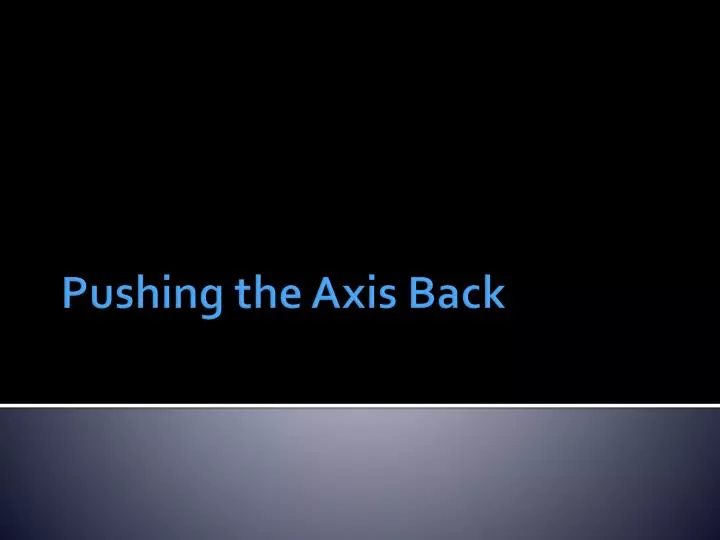The image is the first slide of a World War II-themed PowerPoint presentation titled "Pushing the Axis Back." This slide is predominantly black in the top half, which features light blue Arial text centered and staggered slightly left with the capitalized title "Pushing the Axis Back." A thin white line separates the black top from the gradient gray bottom portion, which transitions from a lighter gray in the center to darker gray at the corners. The overall layout and design suggest a formal presentation, likely intended for an educational setting such as a school or college history class.